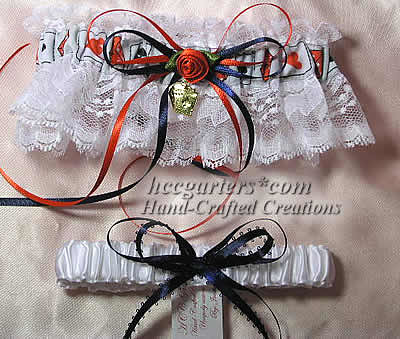The image features two intricately designed garter belts prominently placed in the upper and lower center. Both garter belts boast a delicate white lace ruffle and are adorned with unique, handcrafted decorations. The garter belt at the top is more ornate, featuring a dark blue ribbon, red bows, and a central red rose with green leaves, accented by a gold bell, giving it a playful and flirty appeal. The lower garter belt is simpler but equally elegant, highlighted by two blue string ribbons arranged in a bow. Across the image, a watermark reads "LaceGarter.com Handcraft Creations," indicating the artisanal quality of these distinctive and decorative pieces.